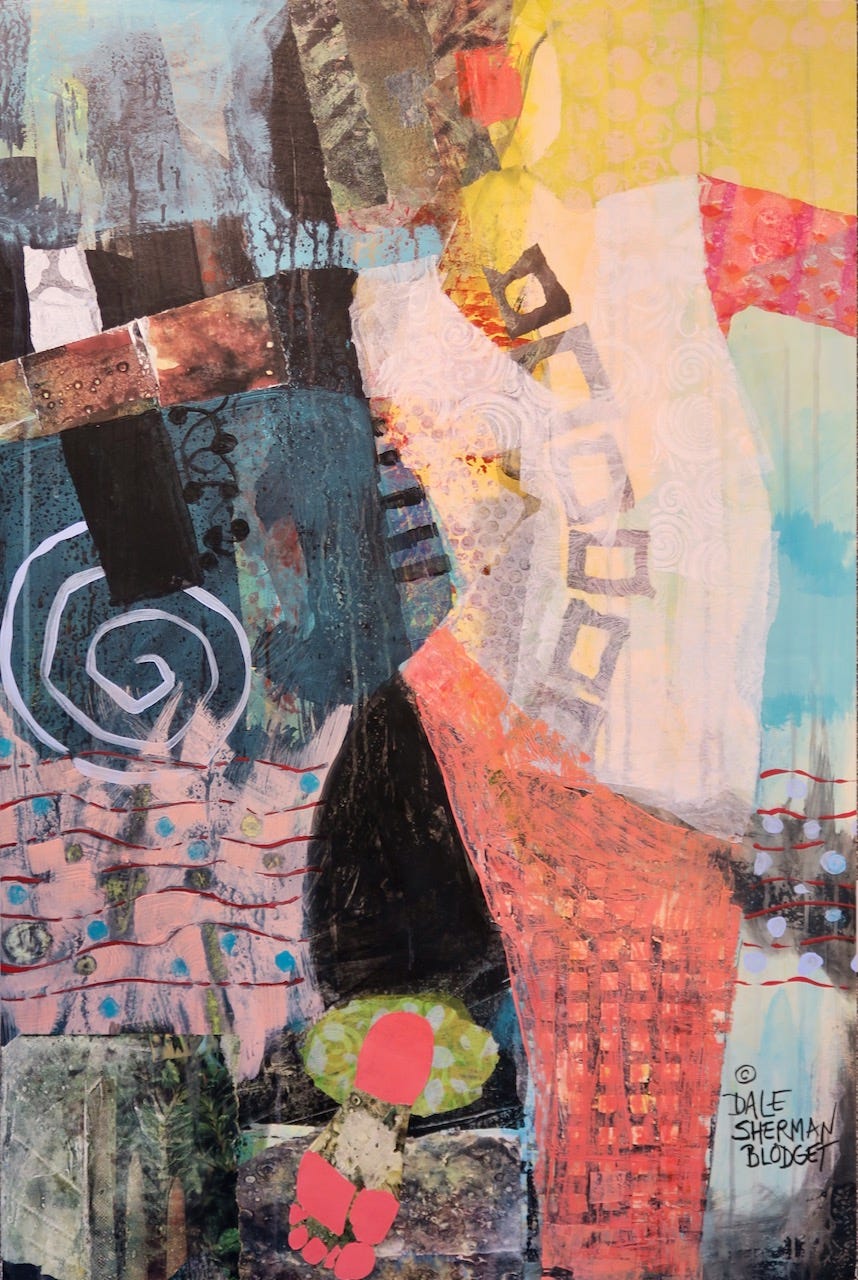The image is a vivid, intricate mural painting by Dale Sherman Blodgett, featuring a woman in a dynamic, dancing pose. The woman's arms are outstretched from her shoulders, with her right arm depicted in black and brown hues, while her left arm is red. She is dressed in a white top and a bottom garment that is delineated into a black right side and a pink left side, though it is unclear if it is a skirt or pants. Notably, she is wearing a pink headphone on her left ear. Her left leg is extended towards the viewer, and her right leg supports her stance.

The background is a cacophony of colors and shapes, including a notable white spiral on top of a blue area under her left arm. To her left, a yellow square transitions into blue hues. The right side, left of the viewer, features blue and black elements, with additional squiggly lines and circles scattered throughout. Below the white spiral, her background transitions into a pink brick wall with a gray square situated at the bottom. The mural captures a sense of vibrant chaos and artistic complexity, emphasized by its dark, contrasting colors. The artwork is signed in black text at the bottom right, noting the copyright and the artist's name, "Dale Sherman Blodgett."